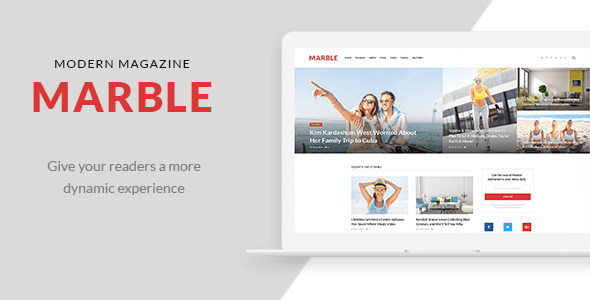In the illuminated image, the left side features a sleek gray background adorned with bold black text that reads "Modern Magazine." Directly beneath, the word "Marble" is highlighted in striking red, followed by a caption in subtle gray text that states, "Give your readers a more dynamic experience." Adjacent to this text is a small image of a laptop.

The laptop screen displays a white background populated with various smaller images. At the top, the word "Marble" appears in prominent white text, accompanied by smaller, unreadable black text. Further down, there is an engaging photograph of a man and woman, both donning sunglasses. The woman points towards something that captivates both their attention.

Embedded within the screen, a red rectangle contains the name "Kim Kardashian" in white text, positioned strategically to stand out. To the side, social media icons are arranged in a neat row: a blue Facebook symbol, a blue Twitter symbol, and a red square with white writing. Additional imagery includes a trio of women seated on a beach, each clad in white sports bras, and a separate picture of a woman wearing a hat, contributing to the mosaic of lifestyle visuals on the laptop screen.